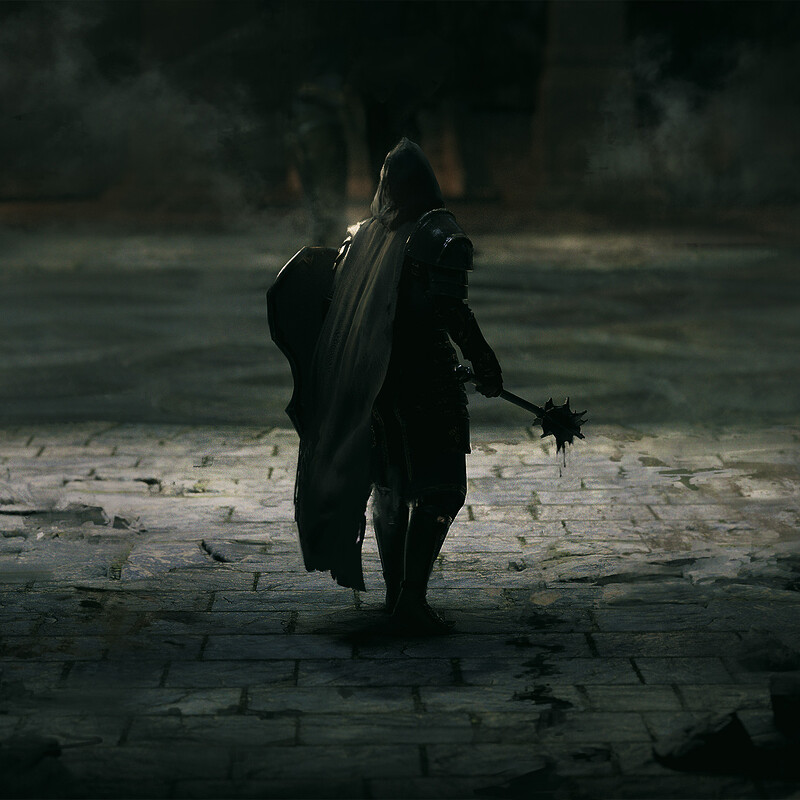In the dimly lit and predominantly grayscale image, a heavily armored knight stands out as the central figure, seemingly caught in a moment of transition. Clad in battle armor and a white robe, he is captured from behind as he strides along an old, cobblestone path that is cracked and overgrown with bits of grass. The knight holds a menacing, spiked mace in one hand, still dripping with blood, and carries a large, imposing shield in the other. A faint light illuminates his immediate surroundings, casting a spotlight on his figure while the rest of the scene fades into deep shadows. The distant background is blurred, revealing only vague shapes that suggest a cliff or a building, enhancing the sense of foreboding and mystery. The overall composition suggests the knight might be heading into battle or retreating from one, adding an element of dramatic tension to the image.